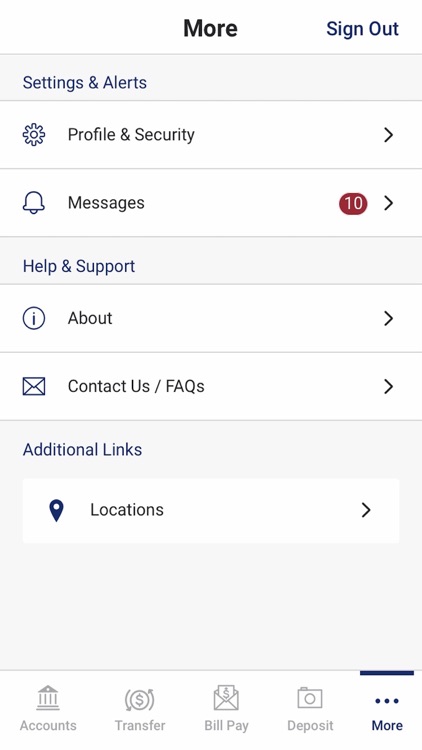Screenshot of a Banking App Interface:

The image captures a screenshot from a banking application, possibly on an Android or iPhone device. The overall background of the interface is predominantly white, with subheadings presented on light gray bars for better distinction. At the top-center of the screen, the word "MORE" is prominently displayed in bold font with initial capitalization. To the right of this heading, the text "SIGN OUT" is visible in a navy-blue font, also in initial caps.

Below the top section, the first gray bar contains the heading "SETTINGS AND ALERTS" in a navy-blue font. Within this section are two selectable options. The first option, denoted by a gear icon, is labeled "PROFILE AND SECURITY" in black font. The second option, distinguished by a bell icon, reads "MESSAGES." To the right of this option, a small red bubble with the white number "10" indicates there are ten unread messages.

Further down, another gray bar titles the section "HELP AND SUPPORT" in blue font. This section contains two options listed in black font: the first is labeled "ABOUT," and the second reads "CONTACT US, FREQUENTLY ASKED QUESTIONS."

This detailed and organized layout ensures users can easily navigate through settings, alerts, and support options.